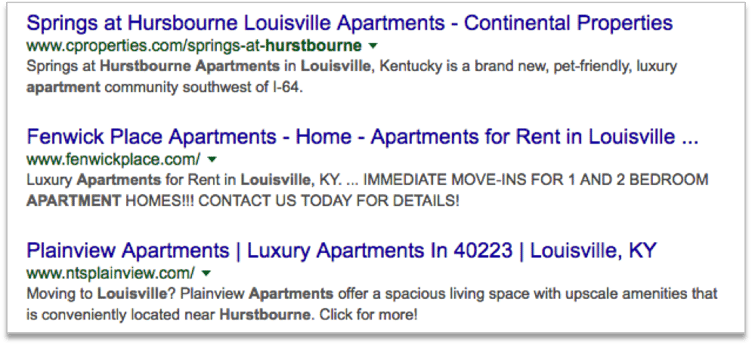A detailed depiction of the Google search result interface is presented within a gray-outlined box, filled with a white background and subtle gray shadows adorning the bottom, left, and right sides. The search results feature three distinct entries:

1. **Springs at Hurstbourne Louisville Apartments – Continental Properties**
   - **URL**: `www.cproperties.com/springs-at-hurstbourne`
   - **Description**: "Springs at Hurstbourne Apartments in Louisville, Kentucky is a brand new pet-friendly luxury apartment community southwest of I-64."
   - The text "Hurstbourne" is bolded, indicating its relevance to the user's search query.
   - **Additional Feature**: A green drop-down arrow is visible next to the URL.

2. **Fenwick Place Apartments – Home – Apartments for Rent in Louisville...**
   - **URL**: `www.fenwickplace.com`
   - **Description**: "Luxury apartments for rent in Louisville, KY... IMMEDIATE MOVE-INS for ONE- and TWO-BEDROOM APARTMENT HOMES. CONTACT US TODAY FOR DETAILS!!!"
   - The emphasis on "IMMEDIATE MOVE-INS" and "CONTACT US TODAY FOR DETAILS!!!" is conveyed through all-caps and multiple exclamation points.
   - **Additional Feature**: A green drop-down arrow is visible next to the URL.

3. **Plainview Apartments | Luxury Apartments in 40223 | Louisville, Kentucky**
   - **URL**: `www.ntsplainview.com`
   - **Description**: "Moving to Louisville? Plainview Apartments offer spacious living space with upscale amenities that is conveniently located near Hurstbourne. Click for more!"
   - **Additional Feature**: No drop-down arrow is visible for this result. 

This clean, precise, and highly detailed caption encapsulates the appearance, content, and specific attributes of each search result within the displayed Google search interface.